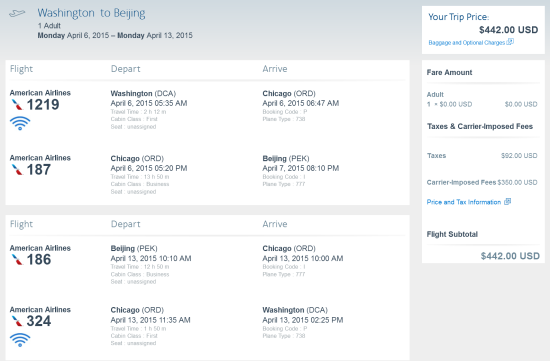### Detailed Caption for Flight Itinerary Image

This image showcases a detailed flight itinerary. At the very top, there is a banner displaying a small airplane logo with the text "Washington to Beijing" in blue, signifying the travel route. This is for one adult, with the departure date set for Monday, April 6, 2015, and the return date on Monday, April 13, 2015.

In the upper right-hand corner, within a white box, the trip's total price is listed as $442 USD. Below this, there is a blue hyperlink text for "baggage and optional charges."

The itinerary is segmented into two main parts: the outbound and return flights, each detailed with flight numbers, logos, and other specifics.

1. **Outbound Flight Details:**
    * **Flight AA 1219:** Departs from Washington, D.C. (DCA) and arrives in Chicago on April 6, 2015. An American Airlines logo featuring blue, white, and red colors with a wing illustration is displayed. This segment has a Wi-Fi logo, indicating in-flight Wi-Fi availability. The cabin class for this leg of the journey is First Class.
    * **Flight AA 187:** Departs from Chicago to Beijing on April 6, 2015, and arrives on April 7, 2015. The aircraft type is a Boeing 777, and the cabin class is Business Class.

2. **Return Flight Details:**
    (Displayed within a separate white box, broken into three rows separating each flight segment.)
    * **Flight AA 186:** Departs Beijing to Chicago. The aircraft is a Boeing 777, with Business Class seating.
    * **Flight AA 324:** Continues from Chicago back to Washington, D.C. The seating for this flight segment is First Class.

On the right-hand side of the itinerary, there's a breakdown of the fare amount. It lists the adult fare along with taxes and carrier-imposed fees, culminating in a flight subtotal of $442 USD.